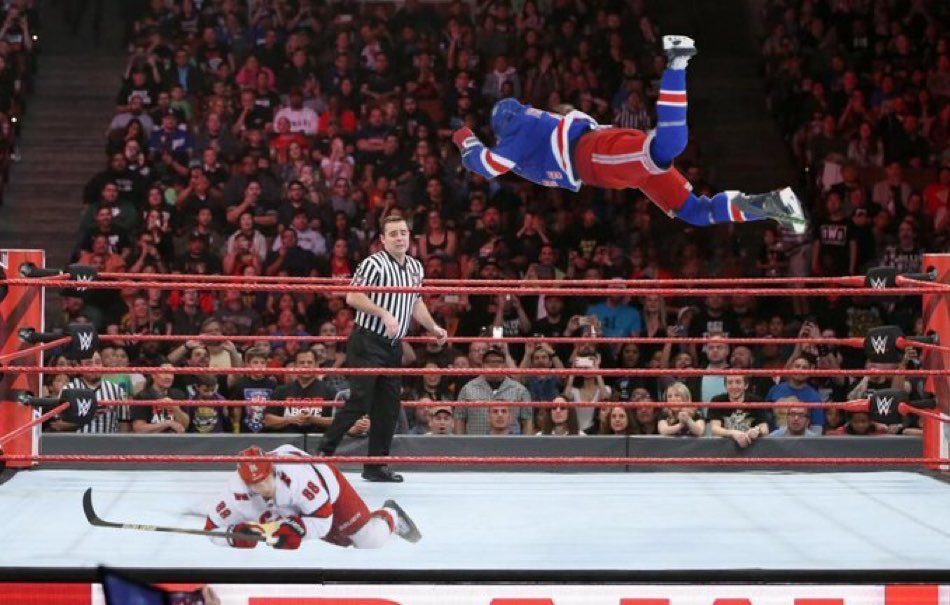In this dynamic image, a wrestling match is staged with an unusual twist: the wrestlers are dressed as hockey players. The central focus is on one wrestler dressed in a red and white hockey jersey and red pants, soaring through the air in an incredible, fully airborne leap. His athletic socks match his jersey, creating a cohesive look. Below him, another wrestler dressed similarly in a red and white jersey and red pants lies on the ground, clutching a hockey stick, adding to the surreal nature of the scene. The grounded wrestler also dons a red helmet, enhancing his hockey player persona.

The action unfolds within a classic wrestling ring, surrounded by an enthusiastic audience. The scene is overseen by a referee in the ring, identifiable by his traditional black and white pinstripe shirt and black pants. Another referee stands on the floor outside the ring, attentively watching the high-flying acrobatics. The crowd's energy and the vivid costumes blend the worlds of wrestling and hockey in a strikingly surreal spectacle.